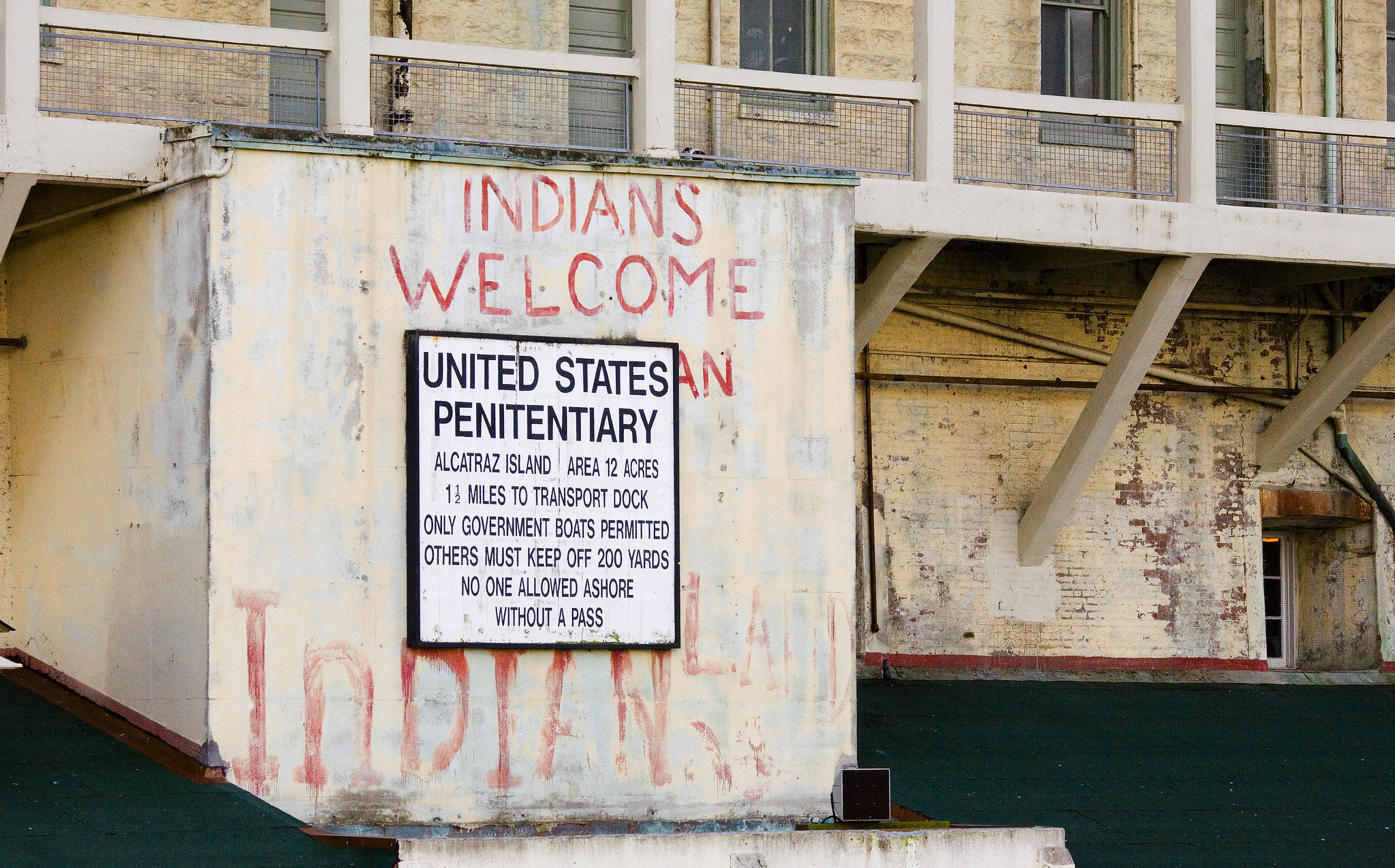This image depicts a historic, weathered facade of an old building, presumably part of the abandoned Alcatraz Island penitentiary. The structure showcases significantly decayed elements, with remnants of white paint barely clinging to the red bricks beneath, especially evident at the building's base where large patches of exposed brick are visible. Architectural features include robust white beams that support an extended porch area, which is safeguarded by a metal fence. The upper sections of the building also display a complex array of wooden beams.

Prominent on the left side of the building is a large, hand-painted sign reading "Indians Welcome," accompanied by other graffitied text that declares "Indian Land," or partially "Indian LA." Official signage below states "United States Penitentiary" followed by details about Alcatraz Island: “Area 12 acres,” “12 miles to transport dock,” “Only government boats permitted. Others must keep off 200 yards. No one allowed ashore without a pass.” This stark juxtaposition of official warnings and subsequent graffiti represents the building's layered history, encapsulating its transition from a notorious penitentiary to a symbol of Native American rights activism.